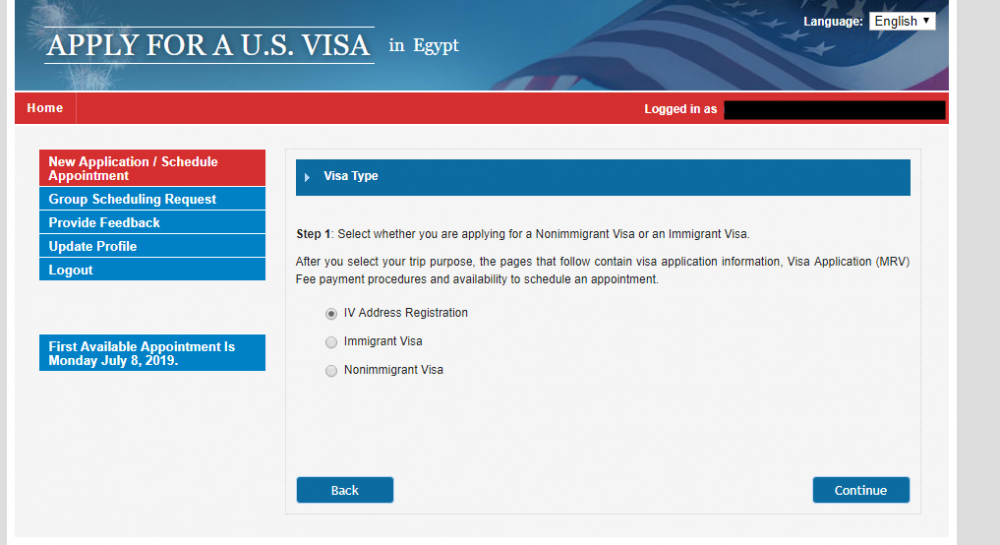The image is a screenshot of a website designed for applying for a U.S. visa, specifically targeting applicants from Egypt. In the upper left corner, the text "Apply for a US Visa" can be seen. The background of the upper left corner features celebratory fireworks, likely to create a welcoming atmosphere. 

On the upper right side, there's an American flag symbolizing the United States. Just below it, the language preference is set to English. A banner near the top of the page reads "Apply for US Visa in Egypt."

Stretching horizontally across the image is a red navigation bar. The bar includes a "Home" link on the far left and a text section that reads "Logged in as," but this is obscured with a black block to protect the user's identity.

Below this red navigation bar, on the left side of the page, there is a vertical menu with several options: "New Application," "Schedule Appointment," "Group Scheduling Request," "Provide Feedback," "Update Profile," and "Log Out."

At the very bottom left corner, it states that the first available appointment is on July 8, 2019. Additionally, on the bottom right, there is a section to select the type of visa, labeled "Visa Type." It indicates this is step one in the application process, where users must choose whether they are applying for a non-immigrant visa, an immigrant visa, or completing address registration.